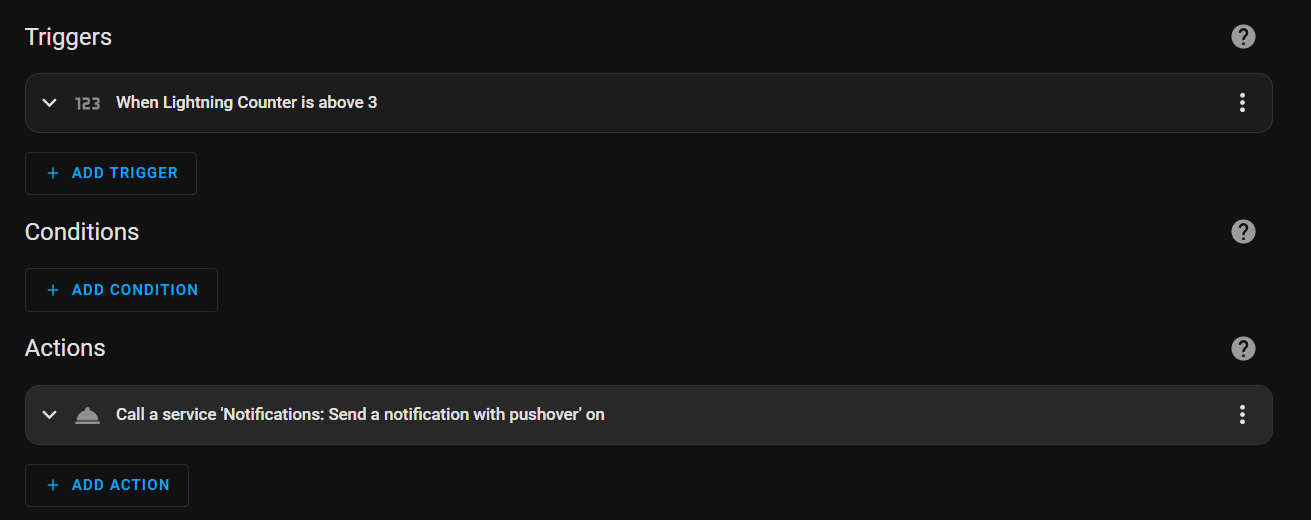This image features a webpage with a sleek black background and white text in its upper left corner labeled "Triggers". Directly below this heading, there's a down arrow icon, the number "123", and a statement indicating "when lightning counter is above 3". Beneath this section, in blue text, is a plus sign followed by "Add Trigger".

Continuing down the page, the section labeled "Conditions" appears in white text. Directly below it is a blue plus sign and the text "Add Condition".

Further down, the section titled "Actions" appears in white text, accompanied by a dropdown box with a bell icon. The dropdown box displays the option "Call a service notification, send a notification, with Pushover on" in white text. A blue plus sign and "Add Action" text follow this section.

On the right-hand side of the page, aligned vertically, are three gray circles each containing a question mark, and two sets of three vertical dots, creating a balanced and organized layout.